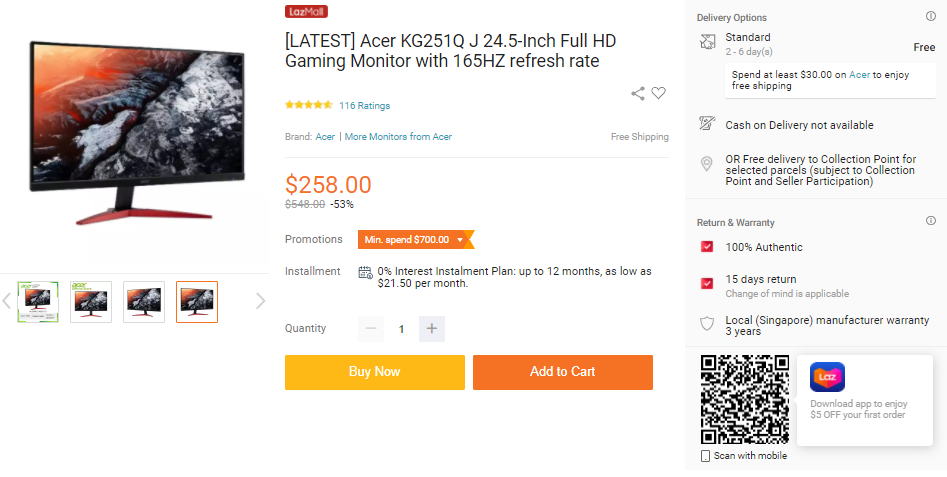This image is a screenshot of an e-commerce product page for a gaming monitor. The page lacks both a header and a footer, leaving the company unnamed. On the left side of the page, there is a photo of the gaming monitor, featuring an abstract image that resembles gray rocks on one side and an orange-shaded sky on the other. 

Centrally located on the page, the product details are prominently displayed. At the top, within gray brackets, the word "Latest" is highlighted. Below, the full product name is listed: "Acer KG25251QJ, 24.5 inch Full HD Gaming Monitor with 165 Hz Refresh Rates."

Directly beneath the product name, the monitor boasts a high customer rating of nearly five full gold stars from 116 reviews, indicating positive feedback from buyers. The price of the monitor is listed in red at $258. 

Below the price, two rectangular buttons offer purchasing options: a yellow "Buy Now" button on the left and an orange "Add to Cart" button on the right. 

On the right side of the page, a sidebar provides additional information, including delivery options. In the bottom right-hand corner of this sidebar, a QR code is visible, likely for quick access or additional product information via a mobile device.